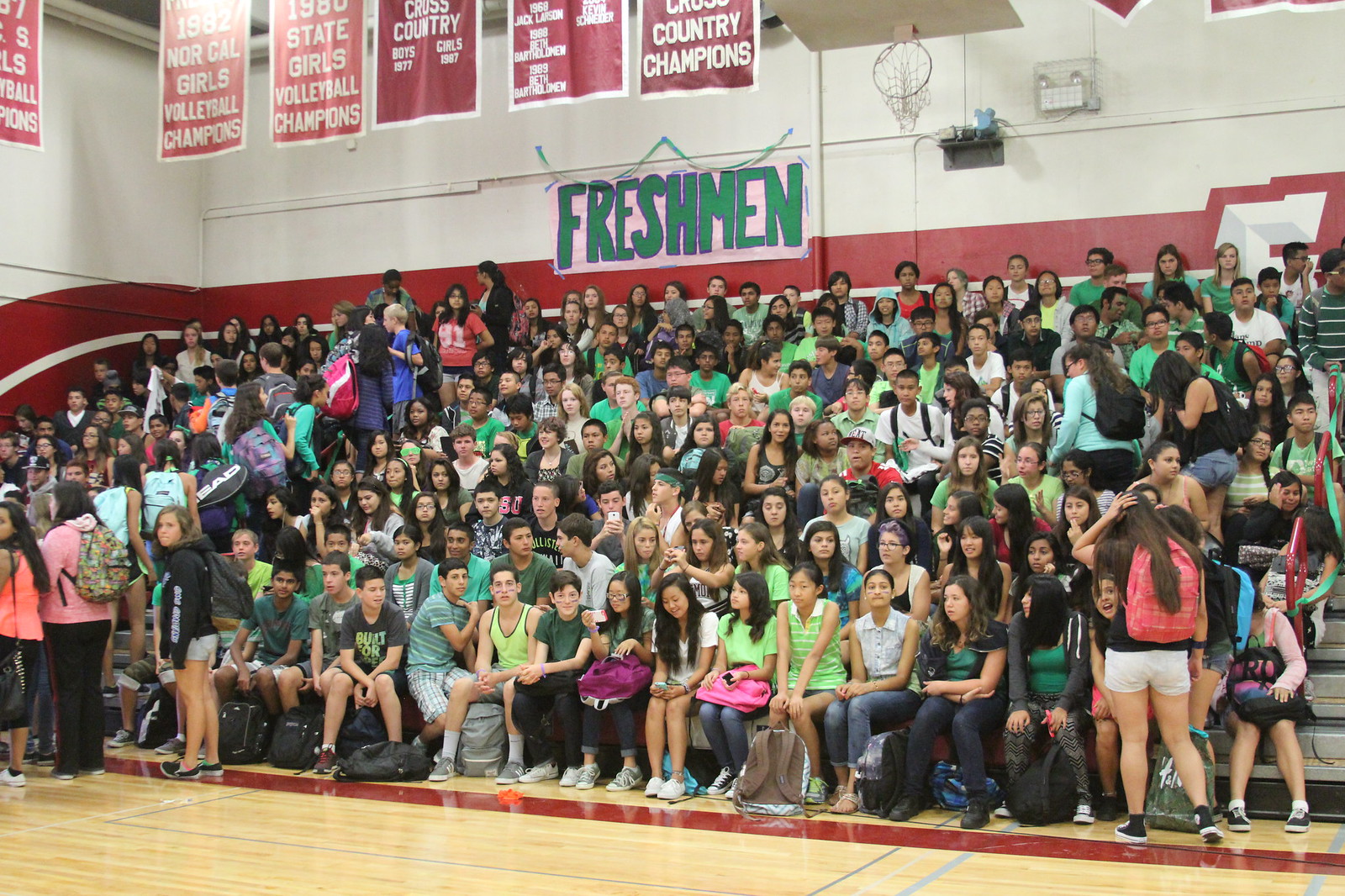The photograph captures a vibrant scene inside a rectangular high school gymnasium during what appears to be a spirit rally. The stands are packed with students, both boys and girls, all of high school age. Most of the students are dressed in either dark green or lime green tops, suggesting these are the school colors. In the foreground, a few students are still walking up the steps, searching for seats. The gymnasium floor gleams with a high-shine light wood grain, typical of such settings.

Above the densely populated bleachers, a large handmade sign with a pink background and bold green block letters reads "FRESHMEN," marking the area where these students are seated. Hanging from the white and red walls and the ceiling are various banners and flags that celebrate past athletic achievements, such as the 1982 NorCal Girls Volleyball Champions and the 1980 State Girls Volleyball Champions, as well as several cross-country accolades. Adding to the sports-centric decor, a basketball hoop is also suspended from the ceiling. The image exudes school spirit and anticipation as students await the commencement of the rally.